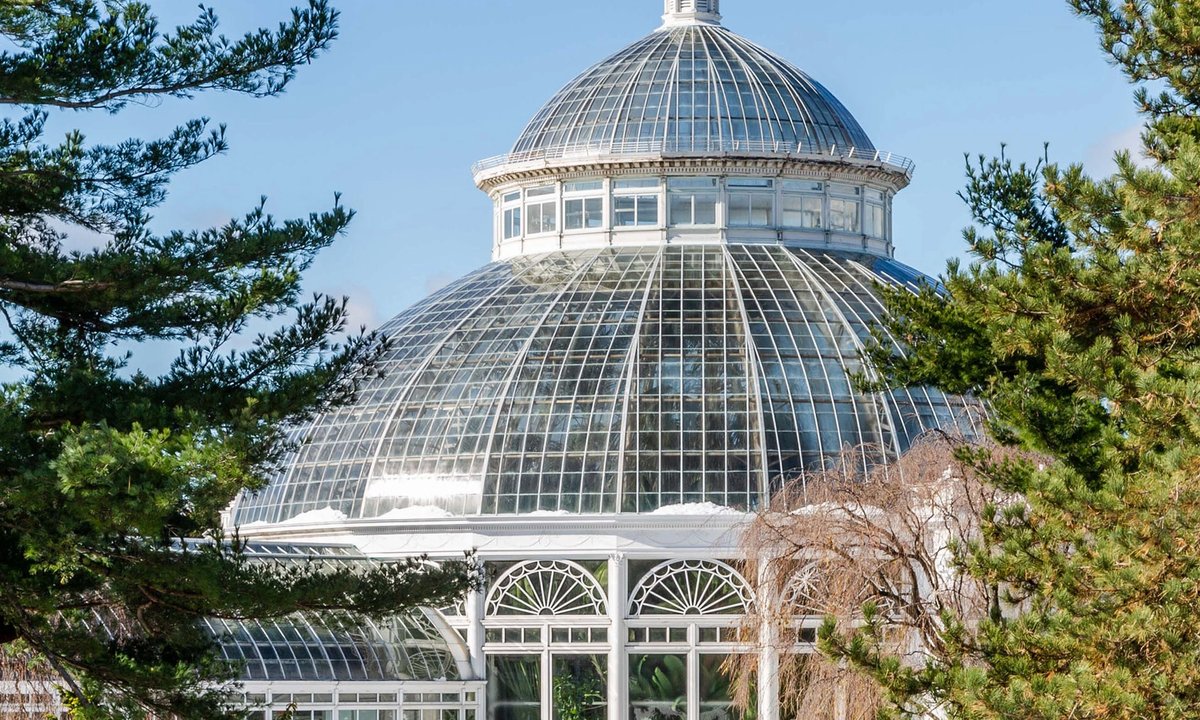The photograph shows an ornate white conservatory or greenhouse with a distinct two-tiered dome structure, set against a clear blue sky. At the top of the building, a smaller dome sits atop a larger central dome, creating a tiered appearance. Surrounding the top dome is a ring of windows, possibly for ventilation or light, and below this central dome, the structure expands outward into another domed section characterized by square patterns of white metal fences and clear glass panels. The ground level of the building features arched windows, adding to its architectural elegance. This intricate structure, possibly dedicated to horticulture or botanical sciences, is surrounded by verdant greenery. Evergreen trees flank both sides of the image, and there is a white fence visible in front and to the left. Inside the glass house, various green plants can be discerned, suggesting it may house a collection of living plants.